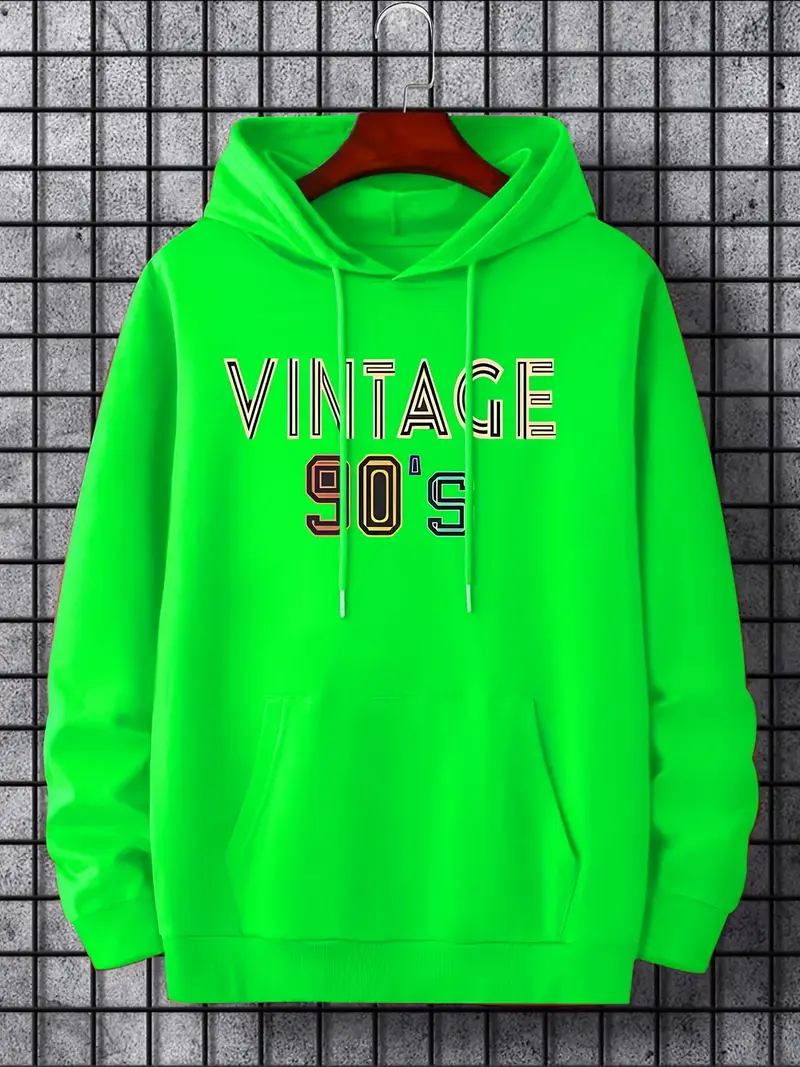The image depicts a vibrant neon green hoodie, prominently marked with the words "Vintage 90s" on the chest. The word "Vintage" is styled in a retro font, appearing white with black details, while "90s" features a mix of orange, yellow, and some green accents, invoking a nostalgic 90s aesthetic. The hoodie, complete with long sleeves, a hood with green drawstrings, and front pockets, hangs from a brown wooden hanger with a silver hook. This hanger is affixed to a metal mesh grid, set against a concrete wall background, enhancing the image's urban feel. The hoodie appears to be an adult size, possibly large or extra-large.